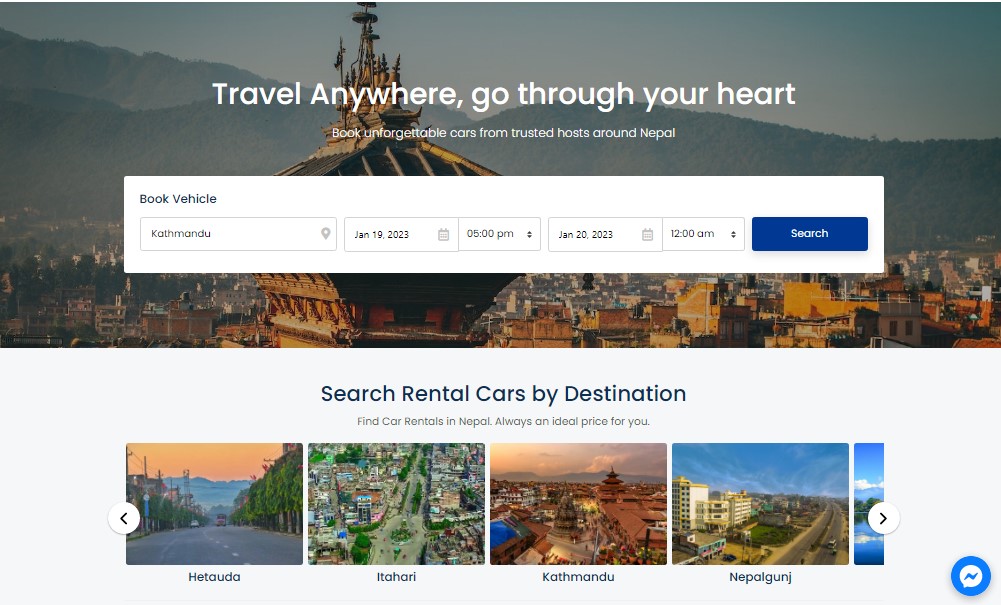This image showcases a section of a travel website dedicated to vehicle rentals. At the very top, a banner invites users to "travel any way your heart desires and book unforgettable cars from trusted hosts around Nepal." Beneath the banner, a vibrant backdrop depicts a bustling cityscape, with an impressive large building in the foreground and majestic mountains under a clear sky in the background.

Centered on this image is a prominent booking pop-up box. The box features a blue "Book Vehicle" button and fields to enter details such as your departure location, departure date and time, return date, and return time. Below these fields is a search bar prompting users to "search rental cars by destination" with the assurance: "Find car rentals in Nepal, always an ideal place for you."

To enhance user experience, there is a horizontally scrolling menu displaying various destinations. The first thumbnail shows a picturesque road flanked by trees and mountains, the second one depicts an urban setting, the third and fourth thumbnails also feature cityscapes, while the partially visible fifth thumbnail hints at another intriguing location.